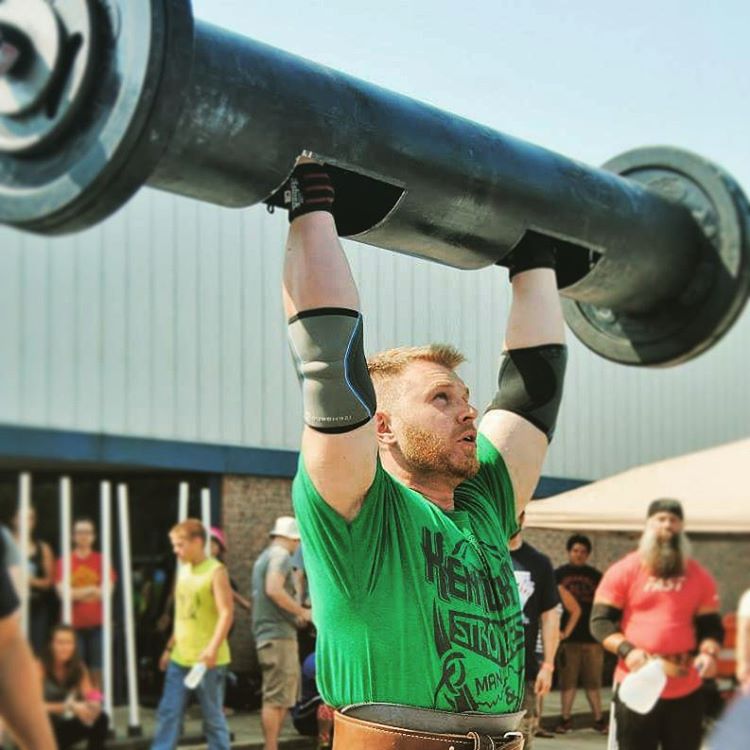A high-resolution photograph captures a muscular man in the midst of a weightlifting event. The man, with short red hair and a closely cropped red beard, is lifting an unusual, heavy black weight. The weight features a thick bar with large round weighted sections on each end and two holes where the man has inserted his arms. Despite the heaviness of the weight, the man appears to lift it effortlessly, as indicated by his calm expression. He is outfitted in a bright green t-shirt emblazoned with text that reads "Strongest," signifying the event. Additionally, he is equipped with black and gray shoulder pads accented with blue highlights, a tan leather weightlifter's belt tightly secured around his waist, black gloves, and elbow supports. In the background, other bodybuilders and spectators, including a bearded man in a red shirt holding a gallon of water, observe the impressive lift.